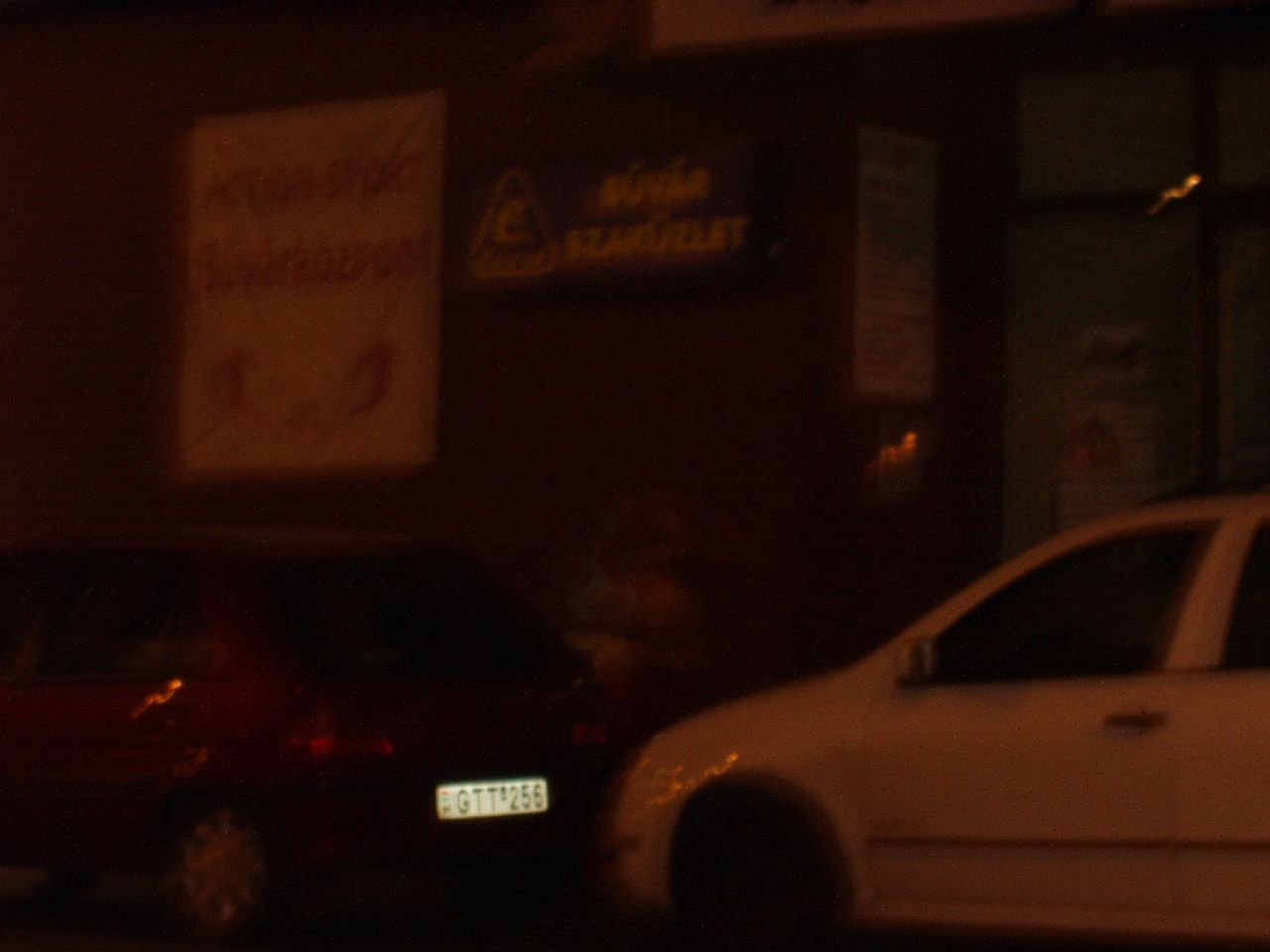The image, taken at night, depicts a street scene featuring two parked cars in front of a building. The right side of the frame shows a white car, but only its front portion is visible. Next to it, a dark red or maroon hatchback car is parked. The license plate of the red car, which reads GTT256, is illuminated by a flash, suggesting a European style. The building behind the cars displays two banners: one is white with red text, and the other darker with white text, both in an unrecognizable foreign language. The image is blurry, and the quality is low, adding to the challenge of identifying finer details.